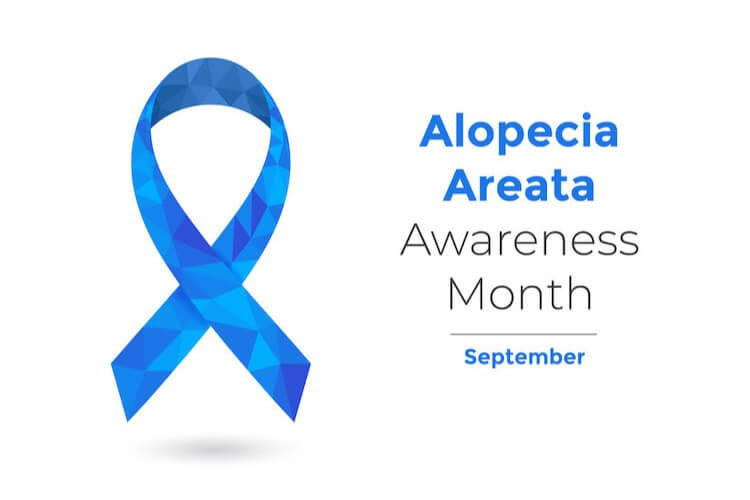This digital rendering features a simple yet impactful design on a white background. On the right side, bold blue text declares "Alopecia Areata," followed by the phrase "Awareness Month" in black. Beneath this, a thin gray horizontal line separates the text, and below it, "September" is written in blue. On the left, a visually striking blue ribbon composed of various shades and triangular segments adds depth and texture, accentuated by a subtle shadow beneath it. The minimalist design, free of any additional background elements, makes this image versatile for use on websites, postcards, letterheads, or other printed materials.